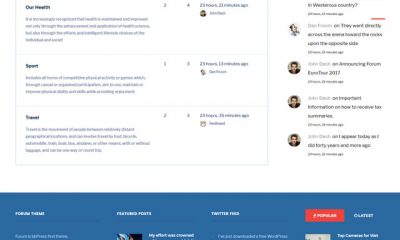The image appears to be a screenshot of a section from a website, showcasing a forum or a discussion board. The background is white with text in black, albeit blurry and hard to decipher. At the bottom of the screenshot, there's a blue bar with white text, though it's too blurry to read clearly. The content resembles FAQs for platforms like Facebook and Twitter. 

On the left-hand side, there's a red button labeled "Popular". Just above this is a label, presumably the title "Our Health," followed by a paragraph that indicates it was posted 23 hours and 20 minutes ago by a user whose profile icon is on the right. The icon depicts a male with short hair, light skin, and wearing a black top.

Below the health section, there's another labeled "Sport," which includes a paragraph posted by another user. Similarly, the "Travel" section follows, with its own user post and profile icon. 

On the right side, the profile icon of the "Sport" post's author is visible at the top, followed by three icons of the person who posted in the "Our Health" section, indicating multiple discussions they're engaged in. The rest of the image remains too blurry to provide further details.